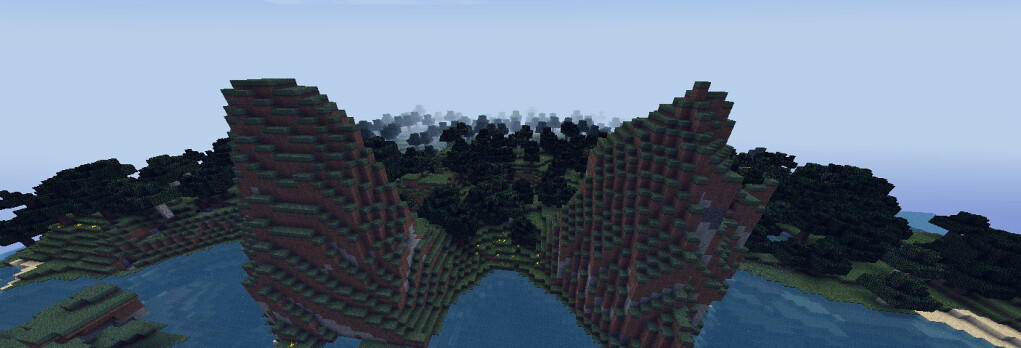The image captured is a Minecraft screenshot presented in a long rectangular landscape format. Central to the image is a striking pixelated terrain featuring two towering cliffs or peaks that bear a resemblance to wings, sloping sharply downwards. These cliffs frame a river flowing beneath, containing varying shades of blue. On both sides of the river, patches of sand are visible. 

Surrounding the foreground terrain, a vibrant field of grass blocks spreads out, dotted with numerous trees showcasing green leaves and brown trunks. To the left side of the image, a small building is discernible among the trees. The background is characterized by distant hills and mountains, which blend into a foggy distance due to limited render or view distance settings. 

The sky above retains a light blue color, with a subtle purple hue on the right side, suggesting either a not-so-bright day or mist shrouding the distant foliage. Though the focus is on the central terrain, the detailed textural elements add rich context to the scene, making it a quintessential snapshot of the Minecraft world.